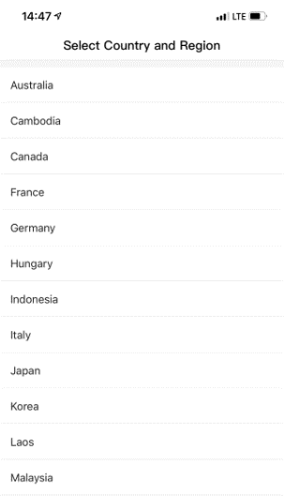The image is a vertically oriented mobile screenshot with a minimalist design on a completely white background. At the very top left of the screen, the time is displayed as 14:47 next to a small triangle icon. On the right-hand side, the battery indicator shows approximately two-thirds charge with a mostly black icon. To the left of the battery icon, the screen displays "LTE" with three out of four black signal bars.

Centered below these status indicators, black text reads "Select Country and Region," with each word capitalized except for "and." Directly beneath this heading is a very thin, light gray horizontal strip extending across the width of the image.

Following the horizontal strip, there is a vertical list of countries, each separated by thin gray horizontal lines. The countries listed from top to bottom are: Australia, Cambodia, Canada, France, Germany, Hungary, Indonesia, Italy, Japan, Korea, Laos, and Malaysia. The same style of thin gray line continues to the bottom of the image, maintaining the clean, organized appearance.